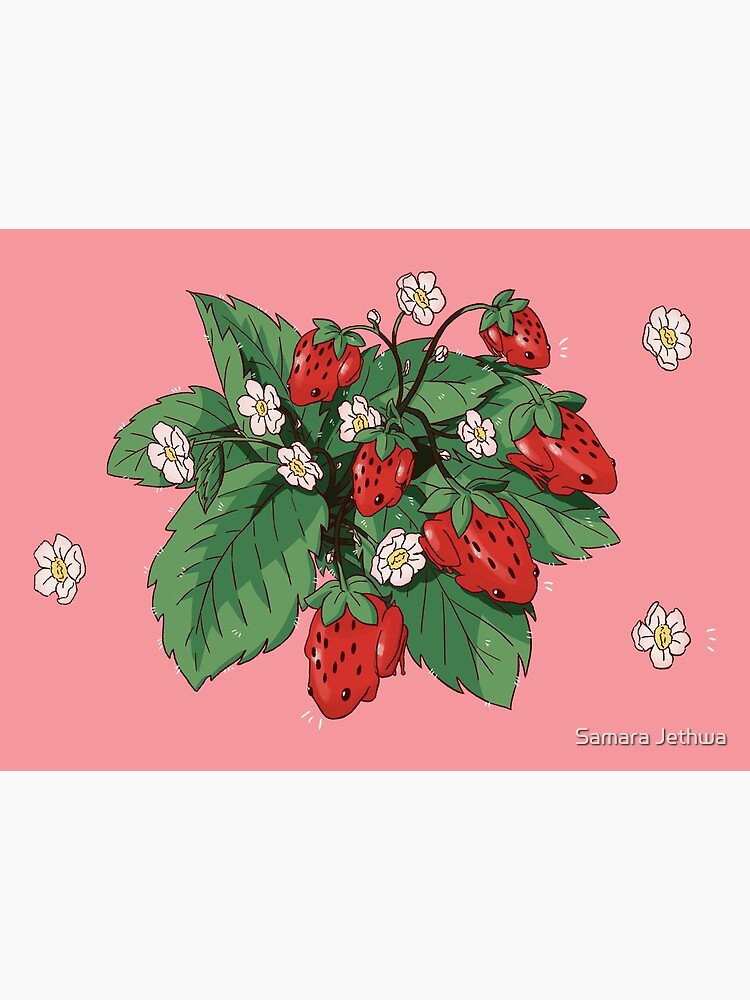This detailed illustration by Samara Jethwa features an imaginative twist on a strawberry plant against a bright pink background. Large green leaves and white flowers with yellow centers characterize the scene. However, in place of traditional strawberries, the focal points are red frogs with black seed-like dots and shiny black eyes, mimicking the appearance of strawberries. The amphibian-fruit hybrids are scattered across the plant, some larger and more prominent, others smaller. Adding to the surreal ambiance are floating white flowers that match those on the plant. The artist's signature, "Samara Jethwa," is displayed in white text in the bottom right corner. Three delicate white lines appear throughout the image, adding to its whimsical nature. This creative artwork seamlessly blends botanicals and amphibians, requiring a closer look to appreciate the clever deception.